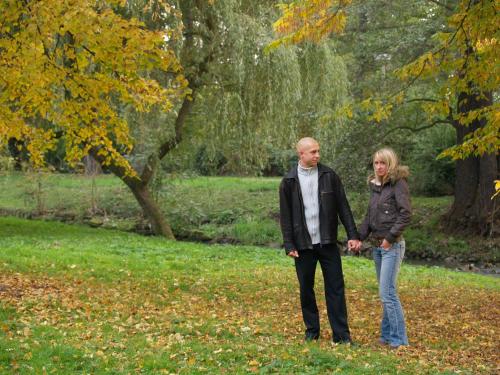In this grainy daytime photograph, a bald man dressed in a black leather jacket over a white turtleneck and black pants stands in a grassy park scattered with autumn leaves. He holds hands with his petite blonde partner, who wears a thick brown jacket with a fur-lined hood and blue jeans. He looks at her affectionately while she gazes into the distance. The couple is positioned in the bottom right of the frame, surrounded by a blend of yellowing trees and evergreen trees that create a picturesque fall setting. Behind the couple, the ground gently inclines into a small hill, dotted with diverse mature trees that enhance the tranquil atmosphere.